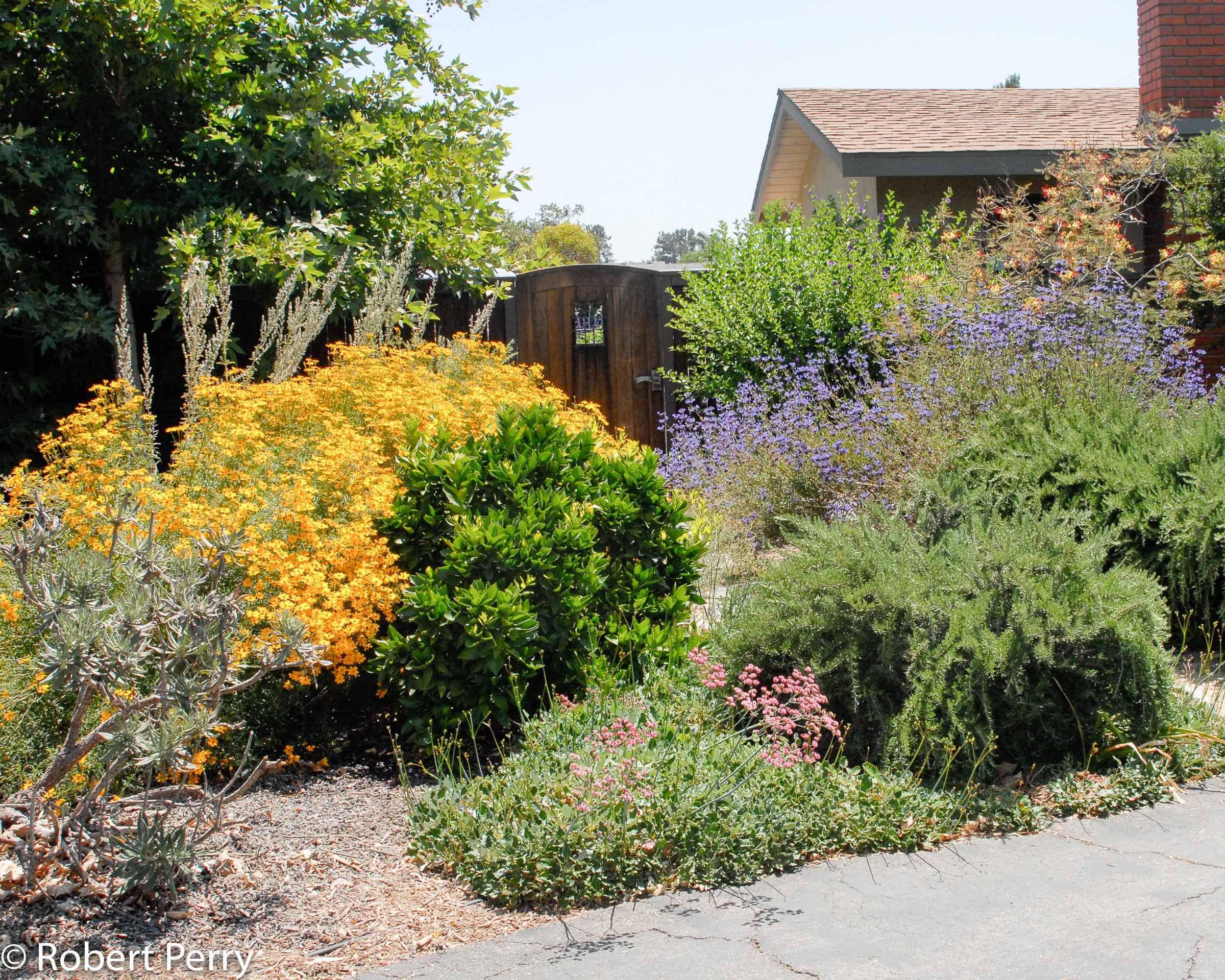The photograph showcases a vibrant and quaint backyard scene on a slightly cloudy fall day. Dominating the left side of the image is a large tree brimming with green leaves, while on the right stands a house with a visible roof and a distinctive red brick chimney. Adjacent to the house is a wooden shed or storage room. In the foreground, a light gray stone sidewalk meanders through a richly planted garden area full of diverse foliage. The garden features a variety of bushes and flowering plants, including gold and purple flowers, vibrant lilacs, and some reddish flowers in the background. Notably, the garden appears overgrown, with lush greenery and colorful blooms creating a wild yet beautiful effect. Completing the image, the bottom left corner bears the white logo and name "Robert Perry," crediting the photographer.